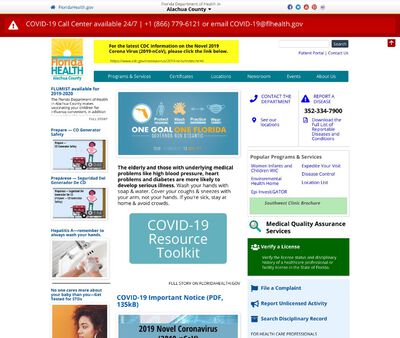The image is a square-framed screenshot of a website with an overall white background. At the very top center, a narrow white banner features the bold black text "Alachua County." Directly below this banner, a red horizontal strip with a triangle alert icon provides a notification. The banner reads, "COVID-19 call center available 24/7" along with a contact number, 866-779-6121, and an email address format ending in "gov."

Below the red banner, on the upper left side within a narrower section than the banner itself, there is the Florida Health sunshine icon. Under this icon, there are a selection of stories, some accompanied by images and titles. In the center of the webpage, a box with the message "One Goal, One Florida" is displayed on a white background. The most prominent and easily readable part of the webpage is situated further down in the center: a light green background with white capitalized text that states "COVID-19 Resource Toolkit." The sides of the images are bordered by a plain white background, framing the central content of the webpage.